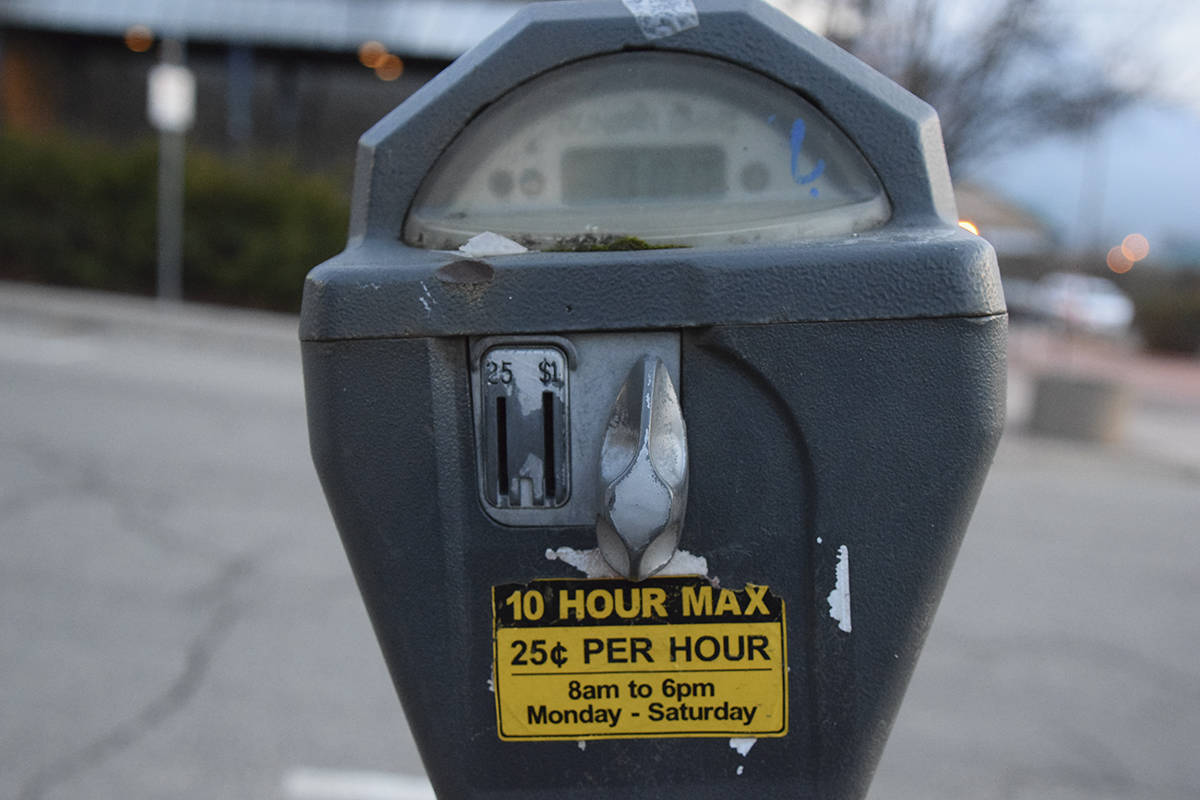The image depicts a worn, old parking meter situated on a blurry city street, possibly during a rainy day. The meter is blackish-blue, made of metal, and shows significant signs of wear, including a faded and scratched surface. The plastic covering the display is hazy and difficult to read, with indistinct numbers visible inside. There's a notable blue mark, somewhat like a backward "J" that resembles fingernail polish, and what appears to be a piece of scotch tape on the top.

At the coin slot area, the instructions for use are partially visible, mentioning the acceptance of 25 cent coins for parking. The yellow sticker under the slot, although chipped and faded, states clearly: "10 hour max, 25 cents per hour, 8 a.m. to 6 p.m., Monday through Saturday," implying that parking is free outside these hours and on Sundays. There's also a dial to set the parking time after depositing the coins.